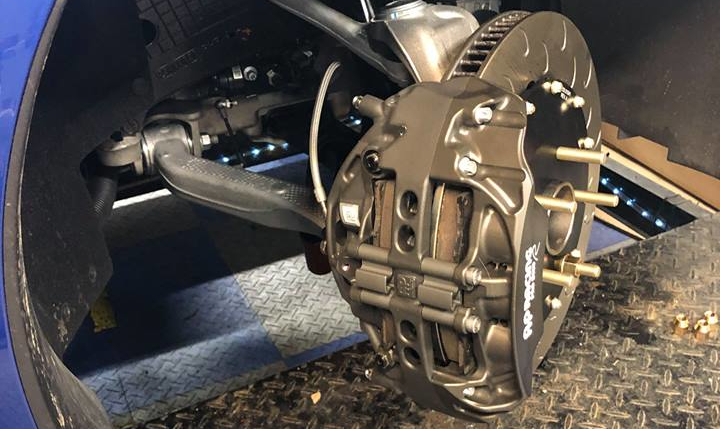This image, taken indoors possibly in a factory setting, showcases a complex machinery setup. Dominating the scene is a large, round, wheel-like gear with short, stubby extensions. This central object has a goldish hue with circular and rectangular indentations, resembling an old-fashioned movie reel. The gear connects to more intricate parts via an arching bar overhead, which reaches into the deeper recesses of the machine. Surrounding the goldish gear, the outer shell of the machinery is blue, while the interior appears darker with black and steel components. Below the main structure, the floor is composed of metal plates characterized by grooves and a textured, raised surface, reminiscent of car rug patterns. The metal flooring varies in color, transitioning from dark and dirty to a cleaner silver section with steps leading into the cavity. To the far right, a panel with a row of bright circular lights and grooved edges can be seen amidst a backdrop of dark, brownish flooring. The intricate and interconnected parts give a glimpse into the inner workings of this sophisticated mechanical apparatus.